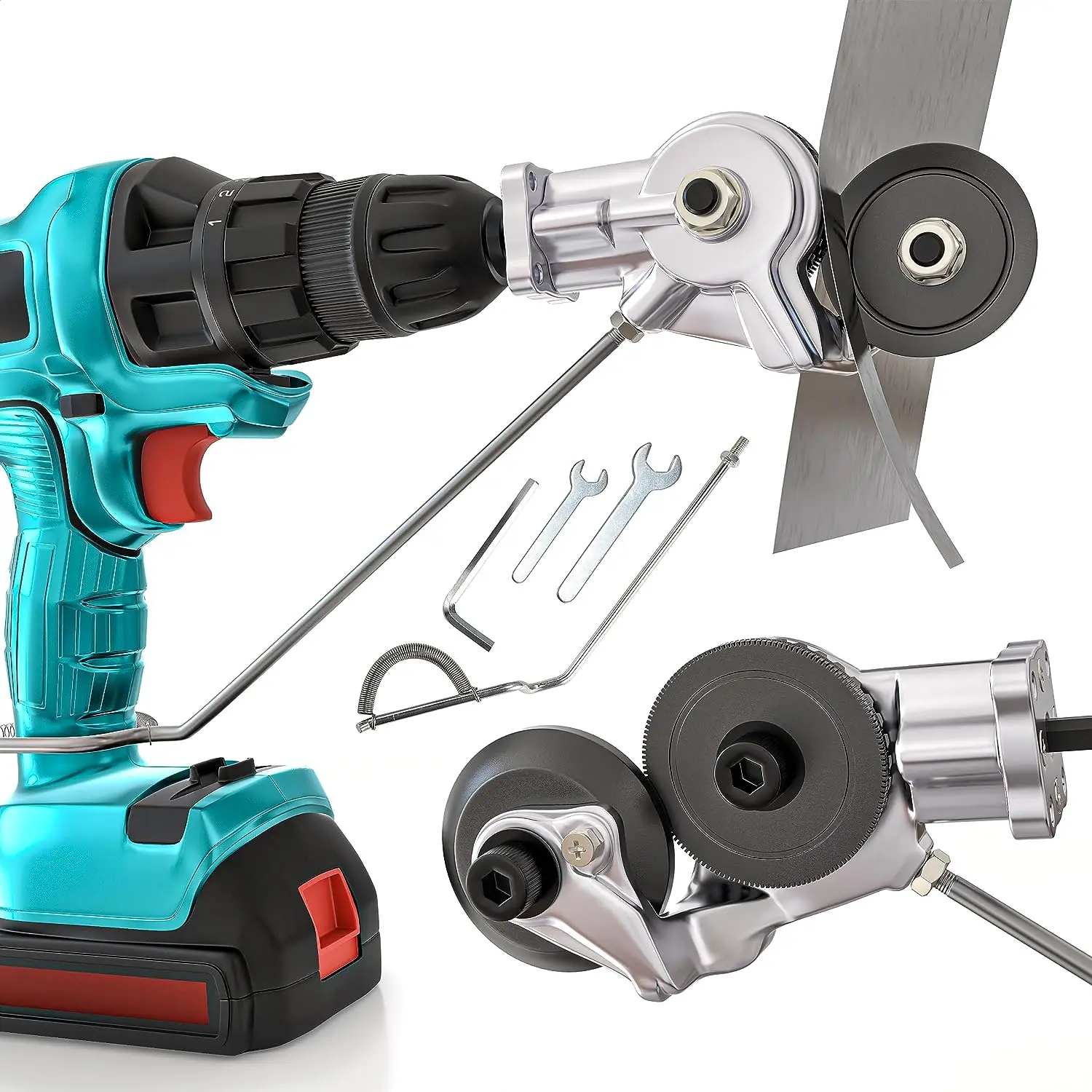The image showcases an electric power drill in a striking teal color with black details and an orange trigger. The drill features a black head designed to hold various bits, with visible numbers indicating adjustable settings. Attached to the head is a chrome device resembling a saw, equipped with a metal plate behind it for user protection. This attachment extends down and secures to the handle, providing extra stability. Below the drill, the image displays an assortment of tools including four wrenches, two with distinctive toothed wheels, and a small Allen wrench. The entire setup is presented on a white background, likely for advertisement or sale, highlighting the drill's vibrant turquoise, black, orange, and silver color scheme.